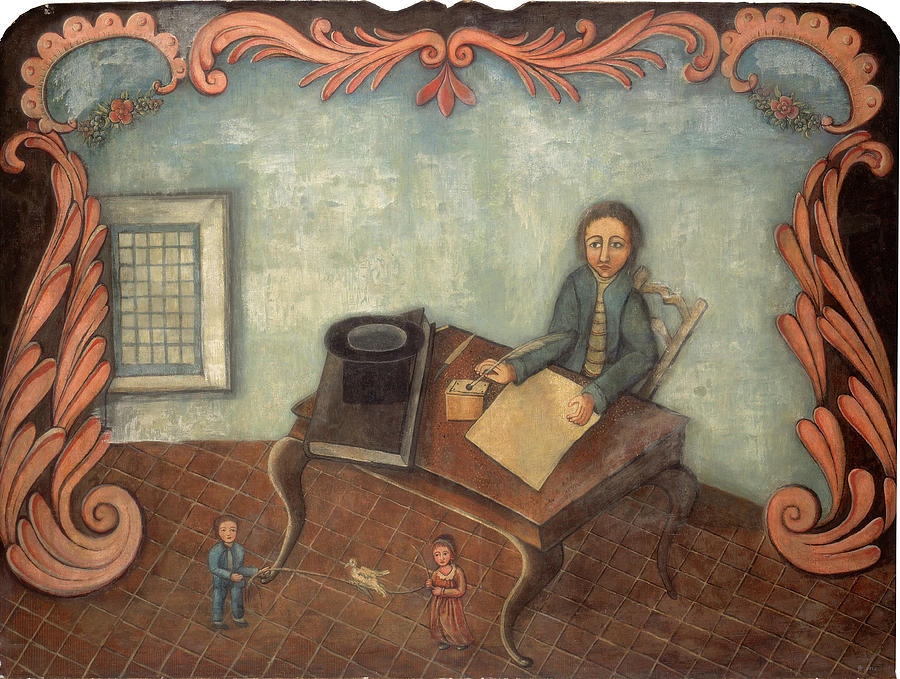The image is an old-fashioned, early American-style illustration, rich in detail but featuring a stylized, flat perspective. It is bordered by ornate, asymmetrical scrolling that may represent a stage. The setting includes a red brick floor and a light gray-blue wall. On the left side of the wall, there is a window with a grid-like design.

In the center of the image, an older gentleman sits at a desk, dipping a quill into an inkwell to write on a blank piece of paper. He is dressed in a blue coat over a gray shirt, with his hair pulled back in an old-fashioned style. On the desk in front of him are his top hat and a book.

Beneath the desk, two small children—out of proportion to the rest of the scene—are playing. The boy wears blue and the girl wears a red dress. They are holding ropes or strings, possibly playing jump rope, with a bird situated in the center of the ropes. The overall image gives off a charming but peculiar sense of scale and perspective.